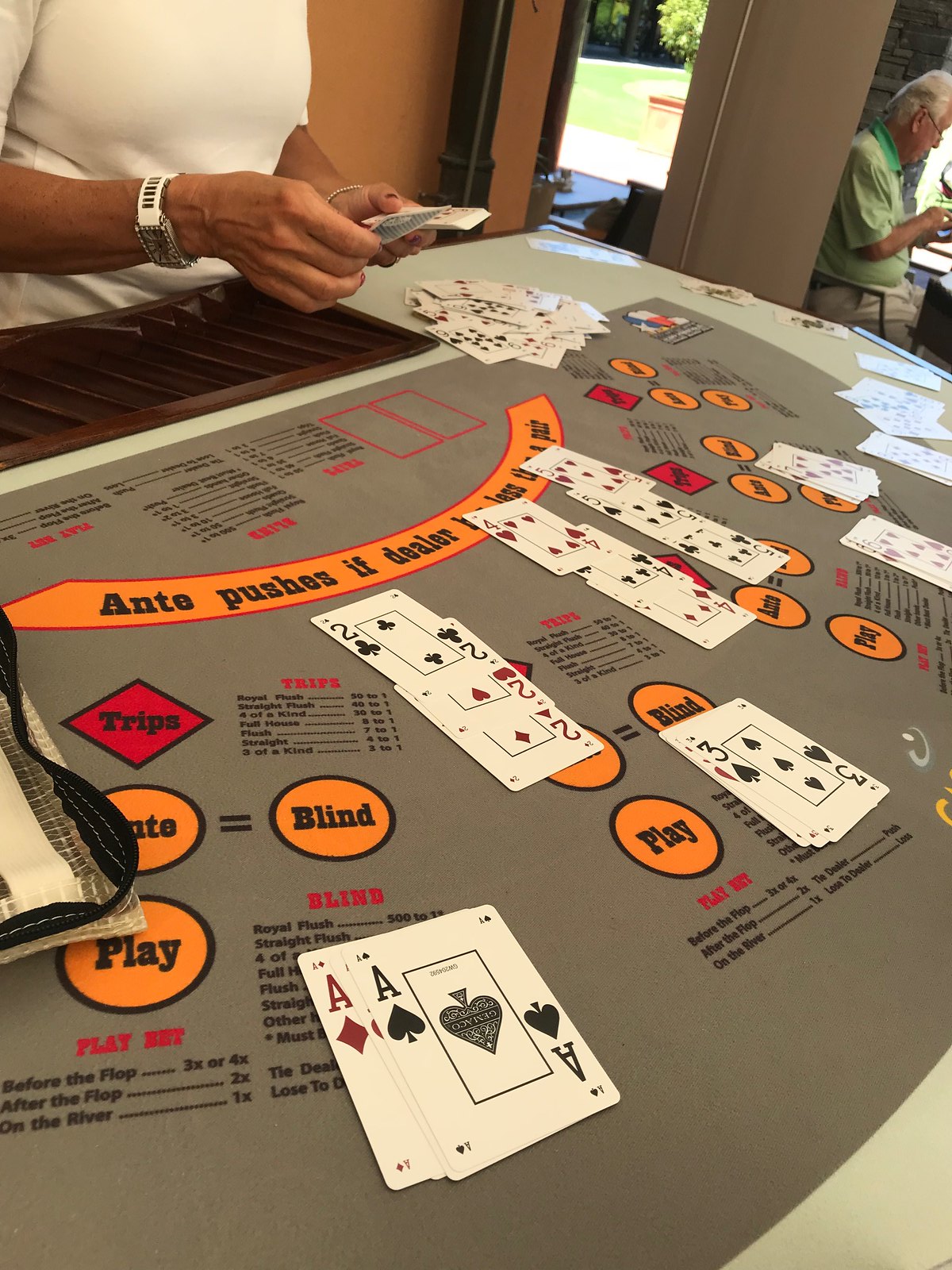This image captures an intricate scene reminiscent of a professional gambling setup, possibly a casino or a private gambling hall. The photograph is vertically oriented and highly detailed, presenting a well-defined foreground and background.

In the backdrop, a beige wall frames an open doorway that leads outdoors. Beyond the door, a sunlit scene reveals a sidewalk bordered by a vibrant green lawn, indicating a bright and pleasant day. To the back right of the image, an older man with gray hair and fair skin stands, partially obscured by a beige wall. He wears a green shirt tucked into khaki pants and gazes downward towards the right, likely focusing on a table out of frame.

The centerpiece of the image is a sophisticated gray card table. This table features a half-circle gray design with lighter gray edges, giving it a polished look. The top left corner of the table hosts a black compartment designed for the dealer to organize her cards and chips. The dealer is a woman with medium brown skin, wearing a white shirt. Her hands, adorned with a white-strapped watch on her right wrist, are busy handling the cards.

The card table itself is adorned with various orange circles and rectangles, contributing to its professional appearance. Among the markings, black text towards the dealer's side reads, "Ante pushes a dealer." Scattered around are orange circles labeled "Play" or "Blind" and several red diamonds with black edges inscribed with the word "Trips." 

Currently, approximately 20 cards are spread face-up on the table. Notably, two aces—an Ace of Spades atop an Ace of Diamonds—are prominently positioned immediately in front of the photographer. Further away lie several pairs of twos and threes, accentuating the detailed and dynamic nature of the scene.